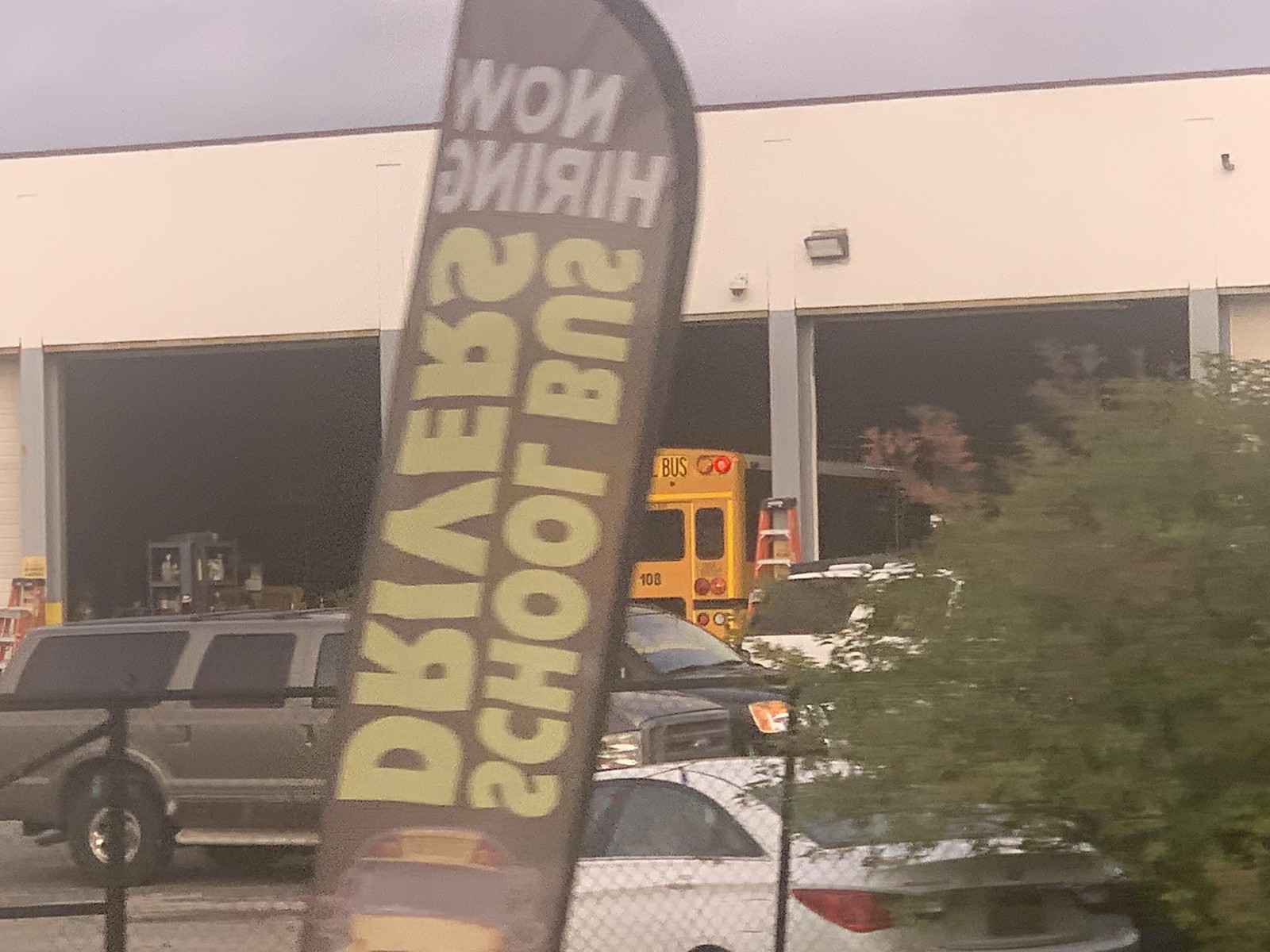This close-up photograph captures a tall, flag-like sign with a distinct, rounded top and rectangular sides. The back side of the sign is visible, but the front-side text can be faintly seen through it in reverse. At the top, in white letters, the sign reads "Now Hiring." Below this, vertical text announces "School Bus Drivers," with "Drivers" aligned to the left and "School Bus" to the right. At the bottom, there is an image of a school bus. 

In the background, a large black chain-link fence separates the sign from a parking lot filled with cars. Beyond the fence, there's a large structure characterized by a row of garages. The photograph reveals four garages, with the rightmost garage door closed. The three central garages are prominently visible, with a school bus parked inside the middle one. Notably, a ladder is propped up against the right side of the last garage visible in the frame.